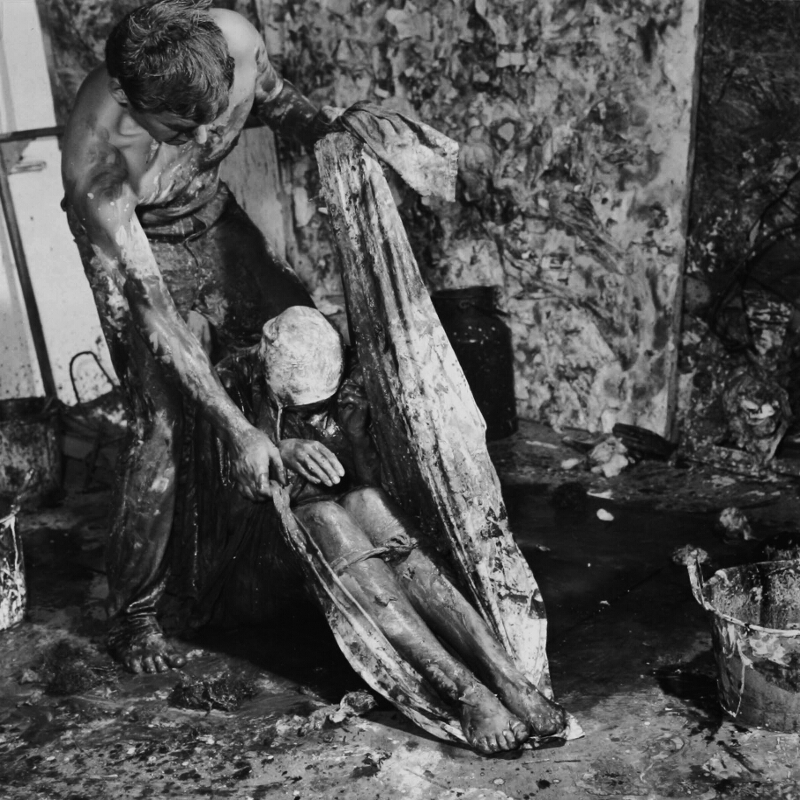This black-and-white photograph captures a gritty, chaotic scene. In the foreground, a shirtless, barefoot man with short dark hair stands amidst a disheveled, muddy area. He is holding a large piece of cloth fashioned into a sling or tarp, which cradles a second figure—a person seated with their head down, only their right hand visible. This person’s legs appear tied together below the knee, hinting at injury or restraint. The surroundings are cluttered with rags, buckets, and what seems to be debris or paint, giving the environment a highly textured, dirty appearance. The background features muddy, paint-smeared canvases and a wall covered in dirt, adding to the overall disarray and somber tone of the image.